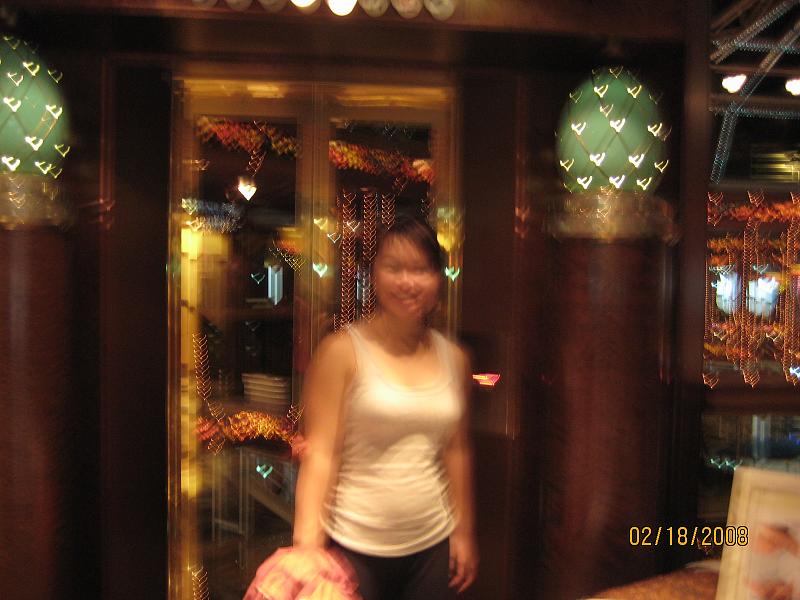In this image, we observe a slightly blurry photograph set in what appears to be a restaurant. The lower right corner of the image displays a date, "02/18/2008," in yellow text. At the bottom of the image, there is a tan picture frame resting on a brown table. 

At the center of the photo, a female figure with brown hair cascading to the side is looking directly at the camera. She is wearing a white tank top and black pants, and she holds a pink object in her left hand. 

The background features a clear doorway that reflects numerous lights, contributing to the overall ambiance. The building's structure comprises brown framing, with the scene further adorned by two green, circular, egg-shaped objects placed on pillars on either side of the central figure.